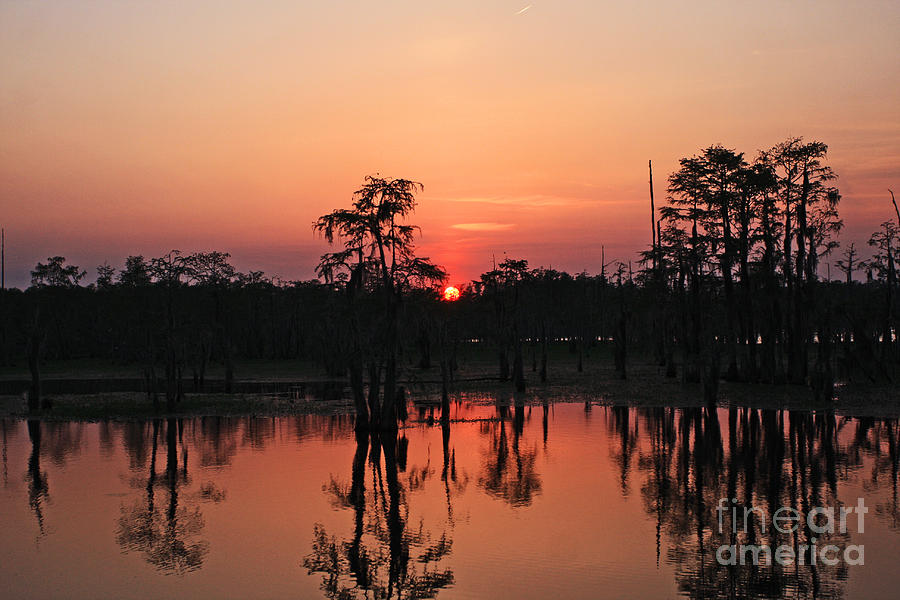A stunning photograph captures the serene beauty of a sunset over a tranquil lake. The sun, a glowing red orb, is partially visible just above the horizon at the center of the image. It casts a pinkish-reddish hue across the sky and waters below, creating a mesmerizing gradient from gray at the water's surface to warm tones higher up. Trees line the shore, their dark silhouettes reflected perfectly in the calm, mirror-like surface of the lake. A dense stand of trees is visible to the right, with a few scattered trees in the middle and left, adding depth to the scene. The sky transitions from the rich colors of sunset to a soft, beige tone towards the top, giving the impression of a fading day. In the lower right-hand corner, the words "fineartamerica" are subtly superimposed in lowercase letters, adding a touch of artisanal branding to this exquisite piece of fine art.